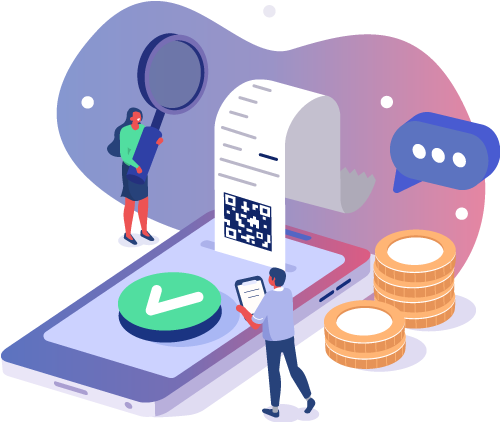The illustration is a whimsical, computer-generated image set against a white background, depicting a cell phone with a stylized, three-dimensional green chip featuring a white check mark on the screen. Emerging from the phone is a white receipt adorned with a QR code, curving gently like an "S." To the left of the cell phone stands an orange-skinned woman in a green long-sleeve shirt and a blue skirt, clutching a large purple magnifying glass that hovers above her head. To the right of the phone are two stacks of yellow-gold coins with white centers, arranged in piles of two and four. Behind the scene, a large, amoeba-like backdrop transitions from purple to pink and is dotted with white spots. Next to it, a bluish-purple speech bubble with three dots hovers above the coin stacks. Below, a reddish-skinned man with dark pants and a light purple shirt faces away, holding a clipboard with squiggly lines, standing in an area with no other distinct elements.